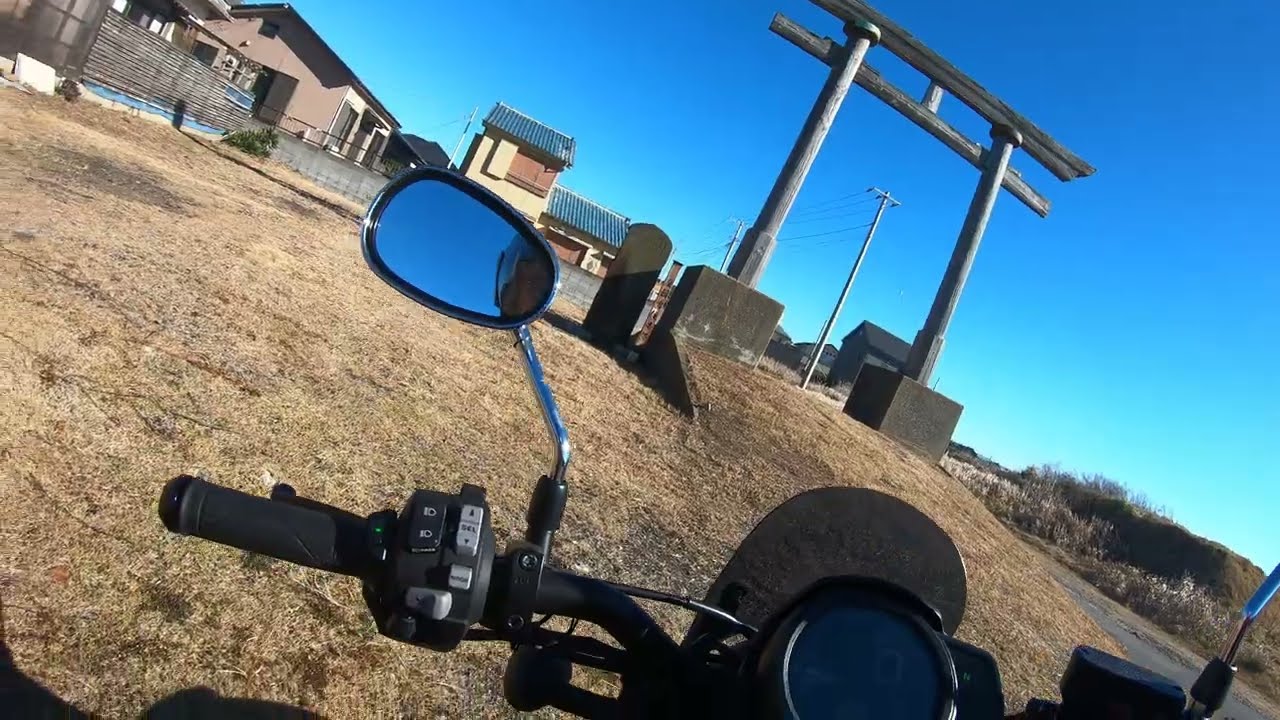The photo captures a first-person view from someone seated on a motorcycle, focusing prominently on the black left handlebar and the small rearview mirror reflecting part of the scene. Slightly to the left, the image shows a rustic setting with dry grass scattered on the ground. A wooden gate is positioned at the top left, while a wooden pillar structure, akin to a ramp or bridge, stands in the middle, slightly elevated. In the background, several houses are visible, blending residential and possibly business structures under a vibrant blue sky. Further details include an archway resembling a Japanese-style structure, power lines, and distant hills, all contributing to the picturesque countryside atmosphere.